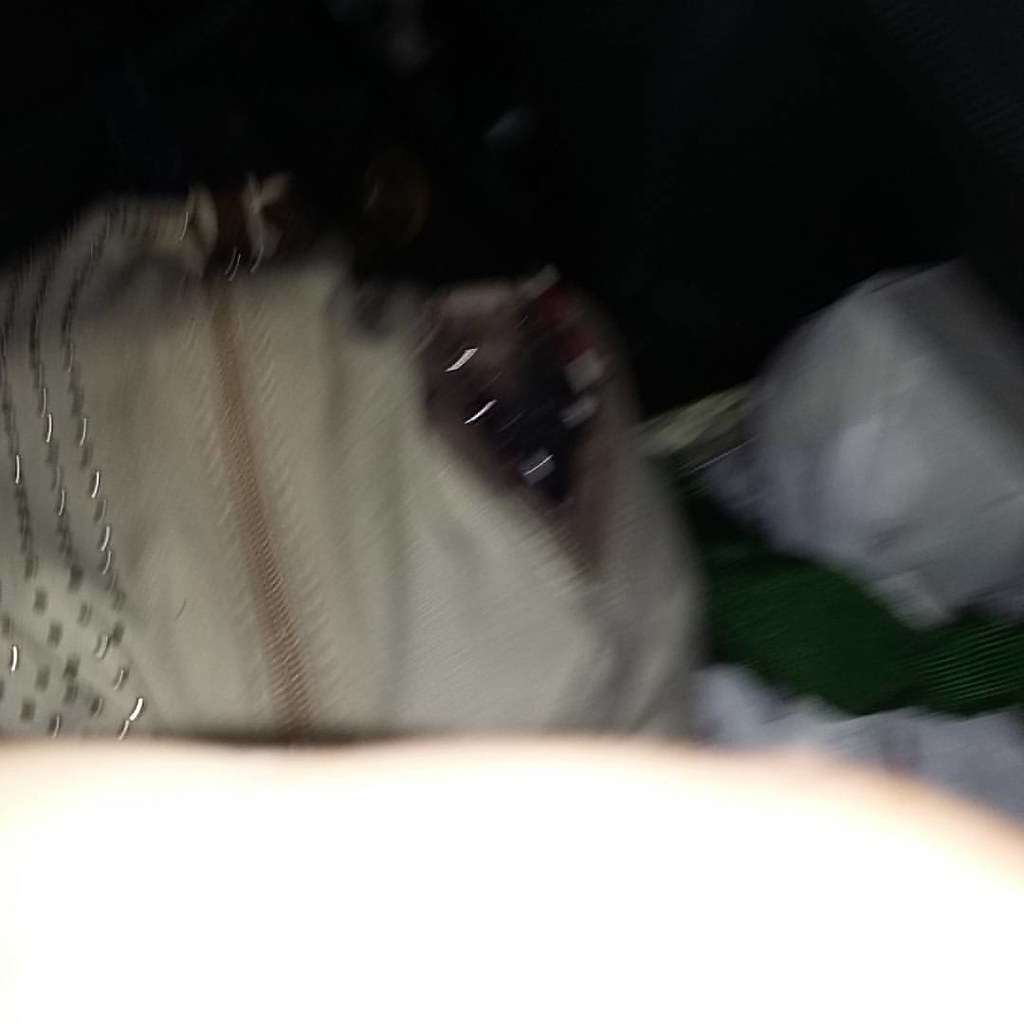The image is a very blurry close-up shot with a predominantly black background, making it challenging to discern specific details. At the center, there is a white article of clothing that initially gives the impression of a bird due to the visible black zipper resembling a beak and one eye-like feature. This white fabric has smooth material adorned with tiny silver beads lined up on the left side. To the right of this white fabric, there is an object that seems tan or beige in color with additional silver details, possibly a piece of jewelry, featuring dark brown and white segments. The zipper is noted as light brown. In front of this, a highly overexposed area appears, likely due to a strong camera flash, and may be part of someone's arm or hand, but it's indistinguishable due to the blurriness. To the left of the white fabric, there are white and dark green sheets with some gold accents. Overall, the image lacks clarity, shrouded by darkness and out-of-focus elements, making it difficult to identify the exact nature of the items depicted.